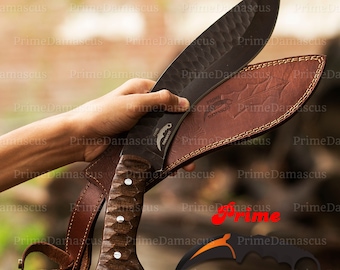A hand, suggesting a Caucasian or Hispanic person based on skin color, is holding a sleek machete knife with a smooth black carbon steel blade. The knife transitions seamlessly into a refined brown handle. Positioned right behind the machete is a brown leather sheath, meticulously crafted to match the shape of the knife. The sheath hints at intricate weaving, possibly featuring the manufacturer's logo. The background behind the knife is intentionally blurred, drawing focus to the detailed craftsmanship of the knife and sheath. In the bottom right corner of the image, the word "prime" is elegantly written in cursive red font. Below this is a small, cartoon graphic of a knife, depicted with black and orange details.